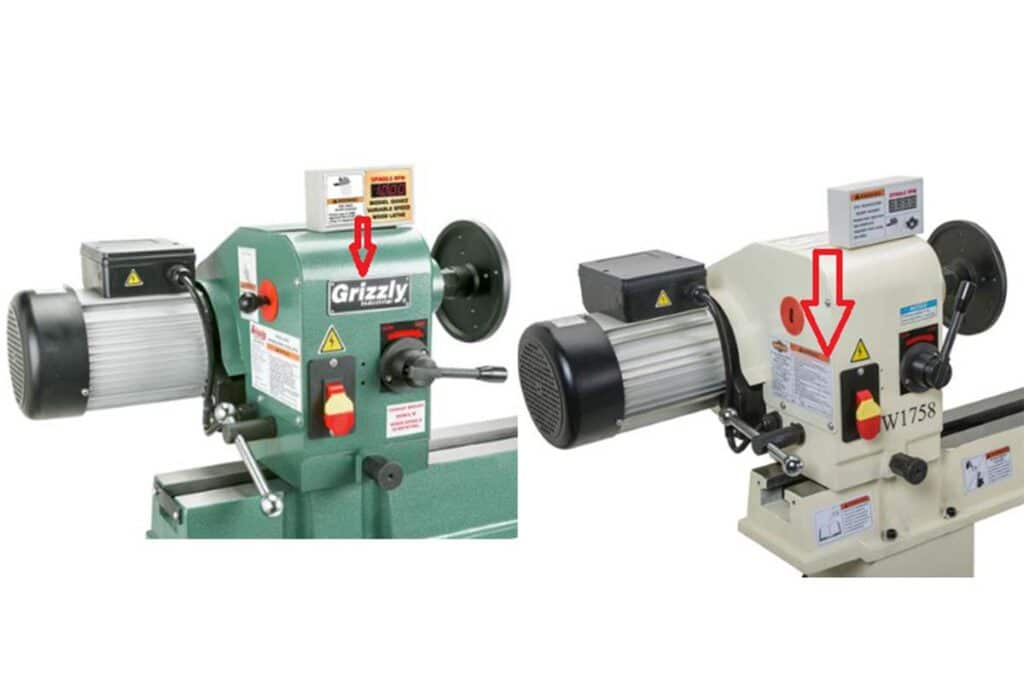This photograph features two nearly identical heavy machines set against a white background, likely used in a specialized workshop. Both devices share the same overall design but differ in color and specific branding details. The machine on the left is green and prominently displays the brand name "Grizzly" in white letters, along with a red arrow pointing to a nameplate. This machine features various knobs and levers, including a cylindrical crank with white grooved lines and a black cap. The right machine is off-white and marked with "W1758" in black lettering, accompanied by a red arrow pointing to a warning sticker. Both machines have rectangular cartridges with printed text on top. Additionally, each device is equipped with different components such as a filter, an electronic box and cord, and a spinning black disc that protrudes from the right side, indicative of their detailed and precise functionality.